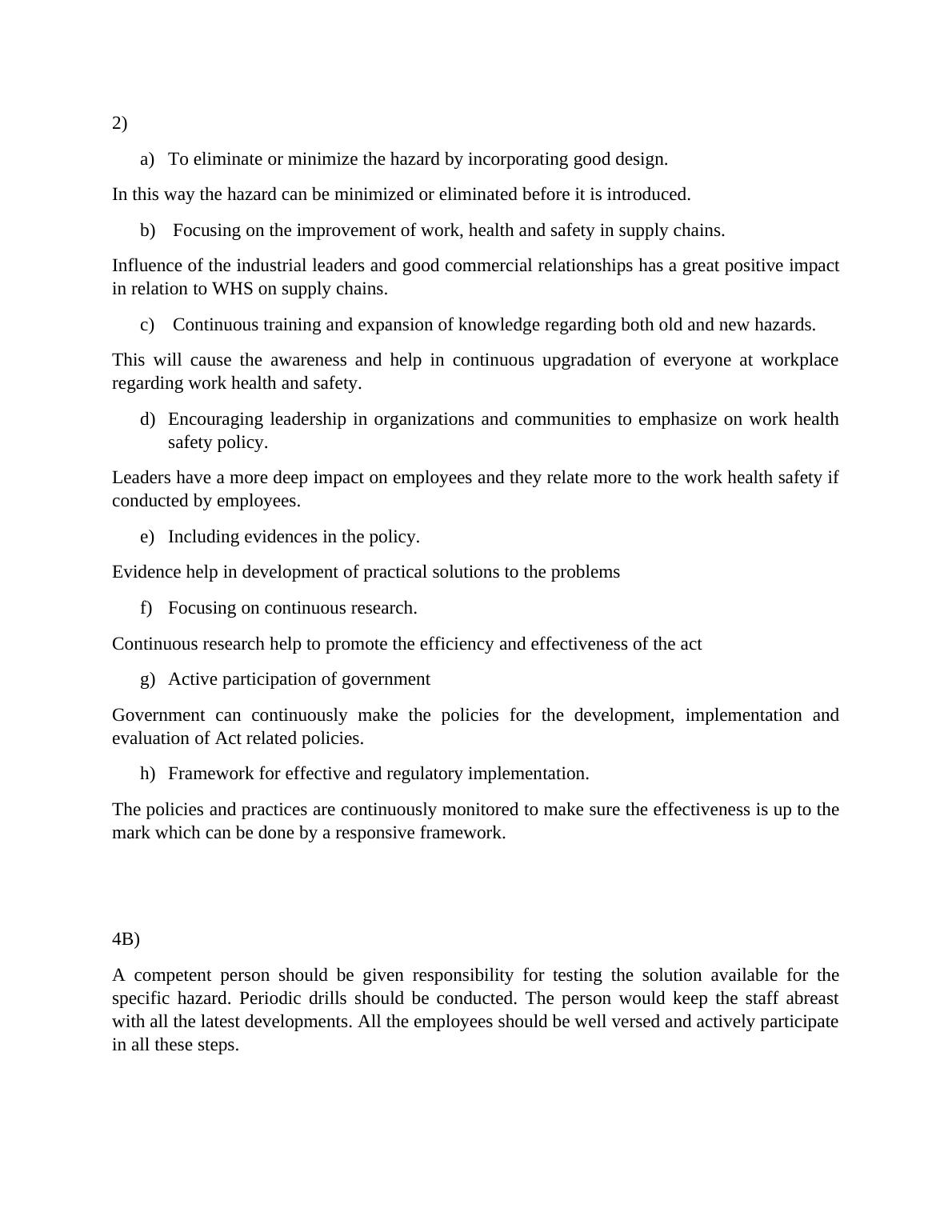This screenshot captures a section of a document labeled with the number "2" which outlines strategic approaches to enhancing workplace health and safety (WHS). 

**A. Eliminate or Minimize Hazards Through Good Design:**
By integrating well-thought-out design principles, potential hazards can be minimized or eliminated even before they are introduced into the workplace.

**B. Improve Work, Health, and Safety in Supply Chains:**
Enhancing WHS in supply chains can significantly benefit from the influence of industrial leaders and fostering robust commercial relationships, creating a positive impact.

**C. Emphasize Continuous Training:**
Ongoing education and training on both existing and emerging hazards ensure that all workplace individuals remain consistently updated and informed about best WHS practices.

**D. Encourage Leadership in WHS Policies:**
Promoting leadership responsibilities within organizations and communities to advocate for stringent WHS policies. Leaders' strong support strengthens employees’ commitment to workplace safety.

**E. Incorporate Evidence in Policy:**
Including factual and research-backed evidence in the development and implementation of WHS policies to ensure they are effective and reliable.

Each point emphasizes specific strategies for maintaining and improving a safe working environment, focusing on proactive design, supply chain improvements, continuous education, leadership endorsement, and evidence-based policy-making.